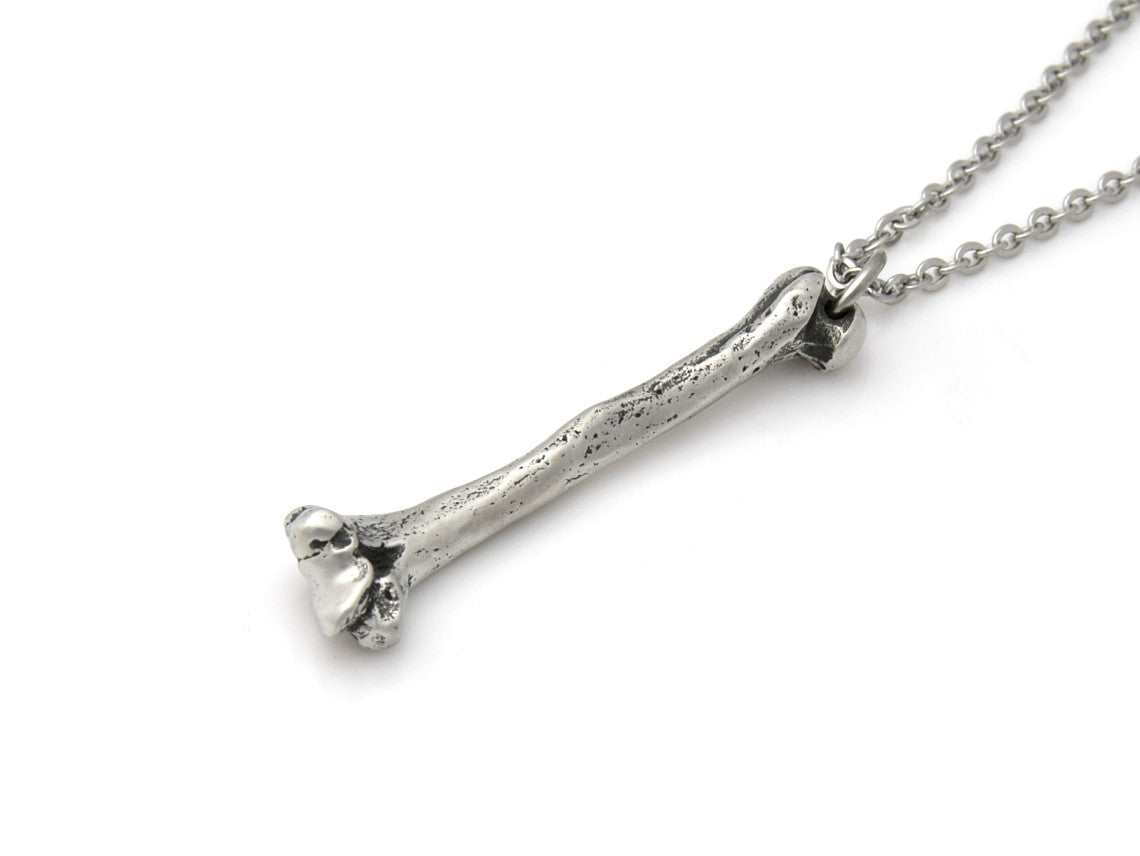This color photograph showcases a rustic, metallic bone pendant, designed to resemble a mammal's femur, attached to a thin, round, silver-colored chain. The bone pendant, pitted with dark gray and black speckles, extends diagonally from the bottom left corner to the top right corner of the image. The top of the pendant mimics the part of the femur that connects to the hip, while the bottom resembles the part that connects to the knee. The plain white background emphasizes the pendant, casting a subtle shadow that enhances its aged, somewhat rusted appearance.